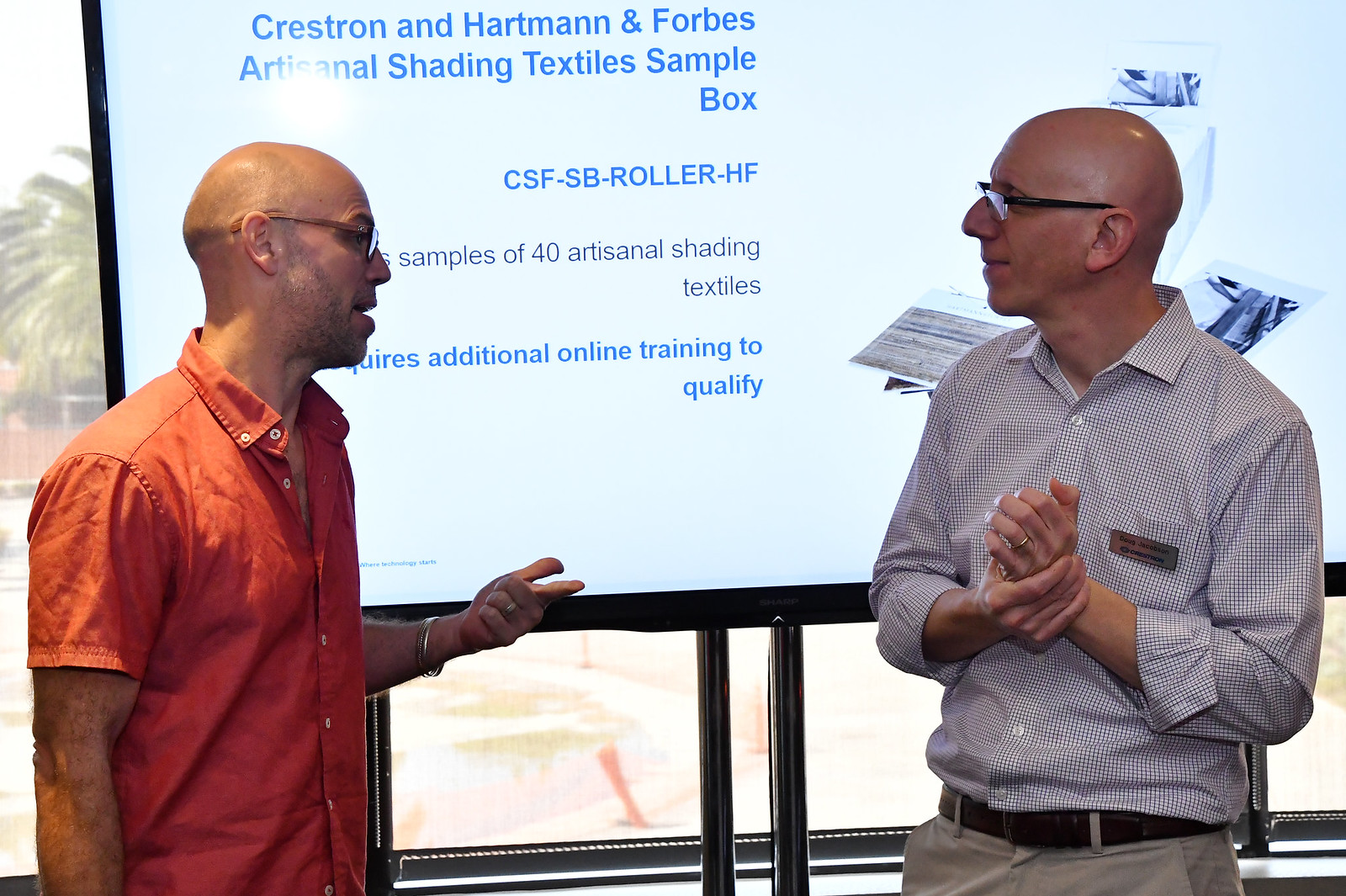In this image, two middle-aged, bald men are engaged in conversation in front of a large electronic screen that features a light blue background. The man on the left is wearing an orange, short-sleeved button-up shirt, without an undershirt, and brown glasses. He sports a stubbled beard, a silver ring, and a bracelet on his left hand. He is gesturing towards the other man with one hand. The man on the right is also bald and bespectacled, donning white glasses, a blue and white checkered button-up shirt, a belt, and gray pants. Both men are wearing wedding rings, indicating they are married. The screen behind them displays a presentation slide with detailed text about "Creston and Hartman and Forbes artisanal shading textiles sample box," mentioning that "CSF SB Roller HF samples of 40 artisanal shading textiles requires additional online training to qualify." In the background, there's a window with some people walking around outdoors, adding depth to the scene.